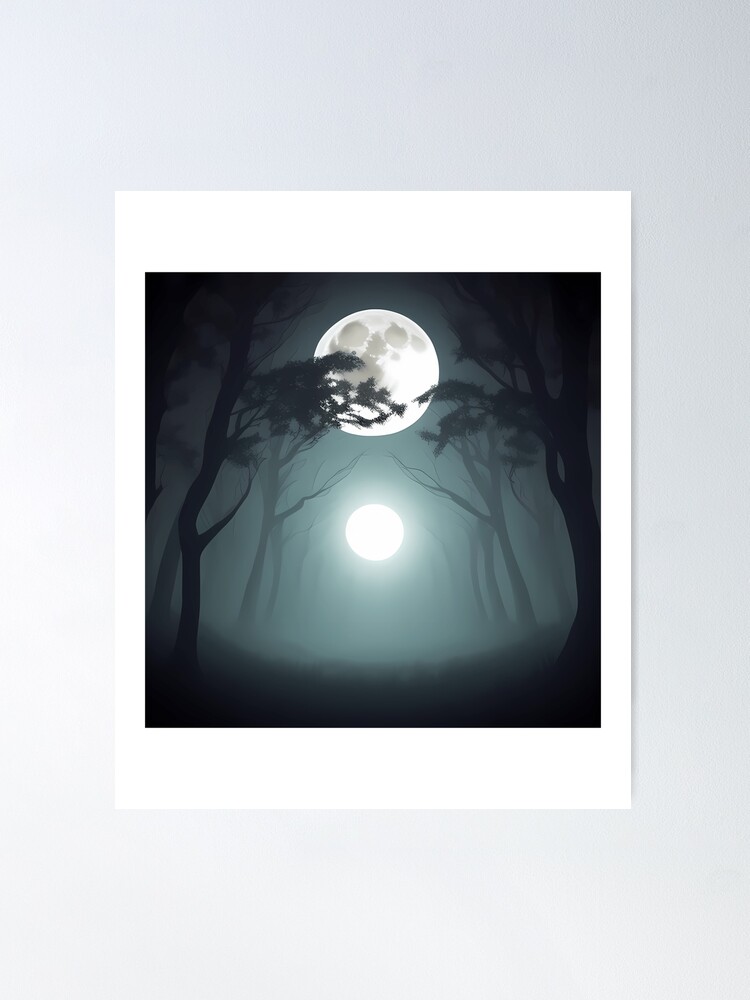This art print evokes a haunting, almost ethereal scene with its dramatic contrasts and eerie details. At the center of the composition is a prominent, craggy moon, high in a gray, misty sky, surrounded by a sparse canopy of black silhouettes of trees that extend towards the moon from both the left and right edges. Below this moon, an enigmatic, bright white sphere - possibly the sun - adds an element of intrigue and confusion, suggesting a surreal conjunction or an impending solar eclipse. The entire scene is depicted on what resembles an old-school Polaroid print, with a white border contrasting against a larger gray background. The top of the image fades into darkness, with fog and mist creating a murky, almost teal hue that enhances the ominous atmosphere. The forest stretches into the distance, shrouded in shadows, amplifying the sense of mystery and symmetry within this arresting night-time tableau.